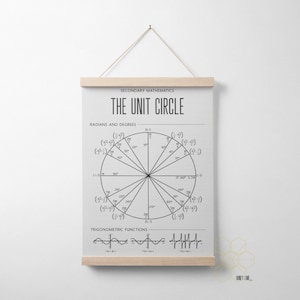The image showcases an artwork-style piece hanging on a light-colored, possibly white or light beige, wall. The piece resembles a poster and is suspended by a string forming a triangular shape fastened with a nail. The poster itself is rectangular, framed by wooden strips at the top and bottom but lacking borders on the sides. 

Prominently displayed on the poster is the title, "THE UNIT CIRCLE" in all caps and black font. Above the title, there appears to be additional text, but it is too small to be legible. Central to the poster is a detailed circular diagram divided into various pie slices of different sizes by black lines, suggesting a mathematical focus – likely depicting trigonometric functions. 

Beneath the circle, the poster features three x and y-axis graphs illustrating sine waves, each accompanied by small, unreadable labels. The piece combines both textual and graphical elements to represent mathematical concepts visually and is thoughtfully placed against a simplistic background to emphasize its intricate details.